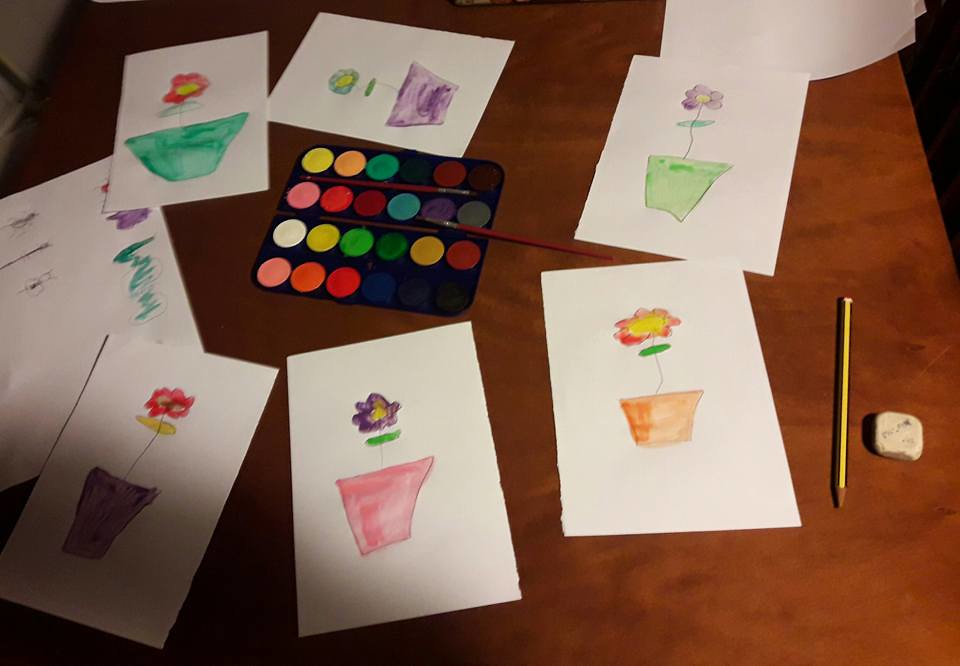The image is a photograph taken from a nearly top-down angle, showcasing a dark-stained wooden table with distinct wood grain patterns. On the table, there are seven small white cards, each featuring a uniquely colored flower pot with a single flower extending from it. Each pot is filled with different colors: two purple, one teal, one green, one orange, and one pink, all varying in size and shape. The flowers have thin, dark-lined stems and simple oval-shaped leaves. The petals are painted in a range of colors, including reds, purples, and greens, all surrounding a yellow center. Towards the right side of the table, there is a green-colored pencil and a small white square eraser. Centrally placed is a color palette with multiple hues such as blues, yellows, greens, reds, blacks, and pinks, accompanied by a small brown paintbrush. The background includes darker cream or off-white shades on the upper left, transitioning to very dark black on the upper right, adding depth and contrast to the scene.